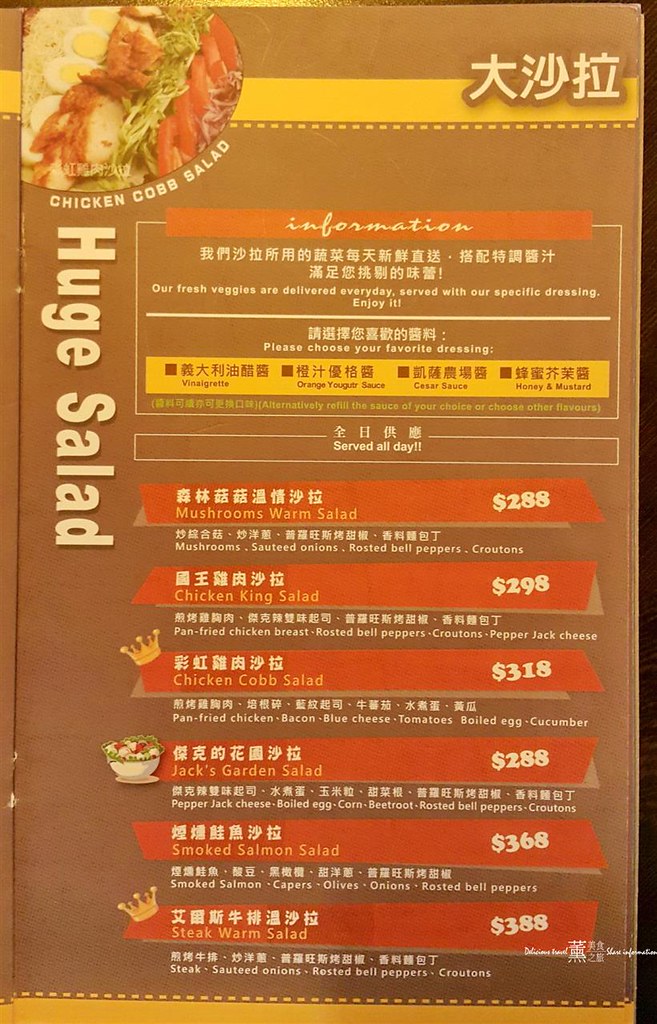The menu board is a bilingual display featuring both English and either Chinese or Japanese text. It includes an actual image of a chicken Cobb salad in the top left corner, showcasing ingredients such as egg, bacon, cheese, tomatoes, and lettuce. Beneath the image, the label reads "Chicken Cobb Salad" with "Huge Salad" written sideways in white lettering. 

Highlighted within red rectangular bars, the board provides additional information. The top bar states "Information," followed by details about the freshness of the vegetables used in the salads and the variety of dressings available: vinaigrette, orange yogurt sauce, Caesar sauce, and honey mustard, all listed in a yellow box. The text underneath, in white letters, assures that the salads are "Served All Day."

Below, the menu lists six different salad options, each within a red box and featuring corresponding prices:
- Mushroom Warm Salad for $2.88
- Chicken Salad for $2.98
- Chicken Cobb Salad for $3.18
- Jack's Garden Salad for $2.88
- Smoked Salmon Salad for $3.68
- Steak Warm Salad for $3.88

Some items are marked with a crown symbol and one with a picture of a salad, potentially indicating special or signature dishes.